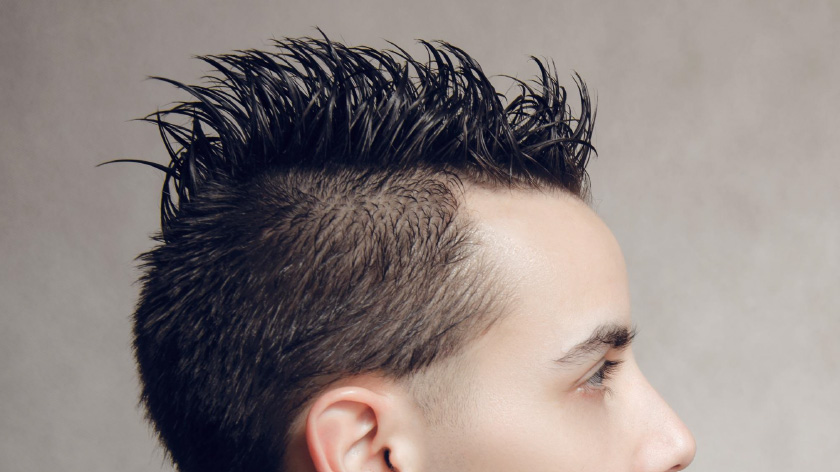The image features a close-up side profile of a young man's head and hair, extending from above the ear down to below the nose. The man has very short, dark hair on the sides, almost shaved. The top of his head features a spiky, gel-applied Mohawk that is about one and a half to two inches tall, appearing shiny and wet. The hairline starts far back, giving the forehead a rounded appearance. His rosy-pink complexion, dark eyebrow, eyelashes, and part of the ear with a visible ear canal are also noticeable. The background is a plain, gradient light to medium gray, offering no distractions from the detailed hairstyle.